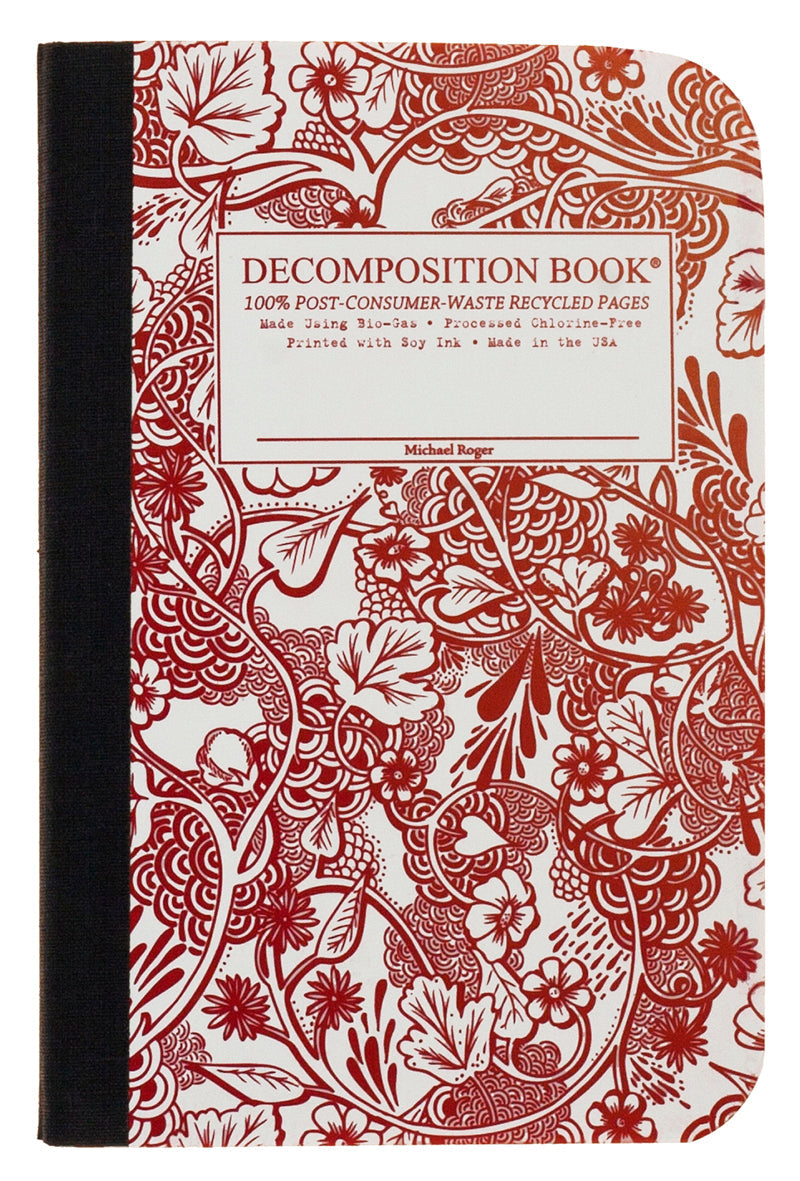The image showcases the cover of a notebook titled "Decomposition Book." The notebook features a black binding on the left side, secured with black tape or fabric. The overall design consists of red floral vines and intricate patterns set against a white background, giving it a traditional and decorative appearance reminiscent of wallpaper or fine china. At the top center of the cover, a white rectangular box contains red text matching the floral patterns, which reads, "Decomposition Book 100% Post-Consumer Waste Recycled Pages made using biogas processed chlorine-free printed with soy ink made in the USA." Beneath this, there is a red line followed by the name "Michael Roger" in red text, perhaps indicating the artist or producer. The detailed and eco-friendly design highlights both aesthetic appeal and sustainability.